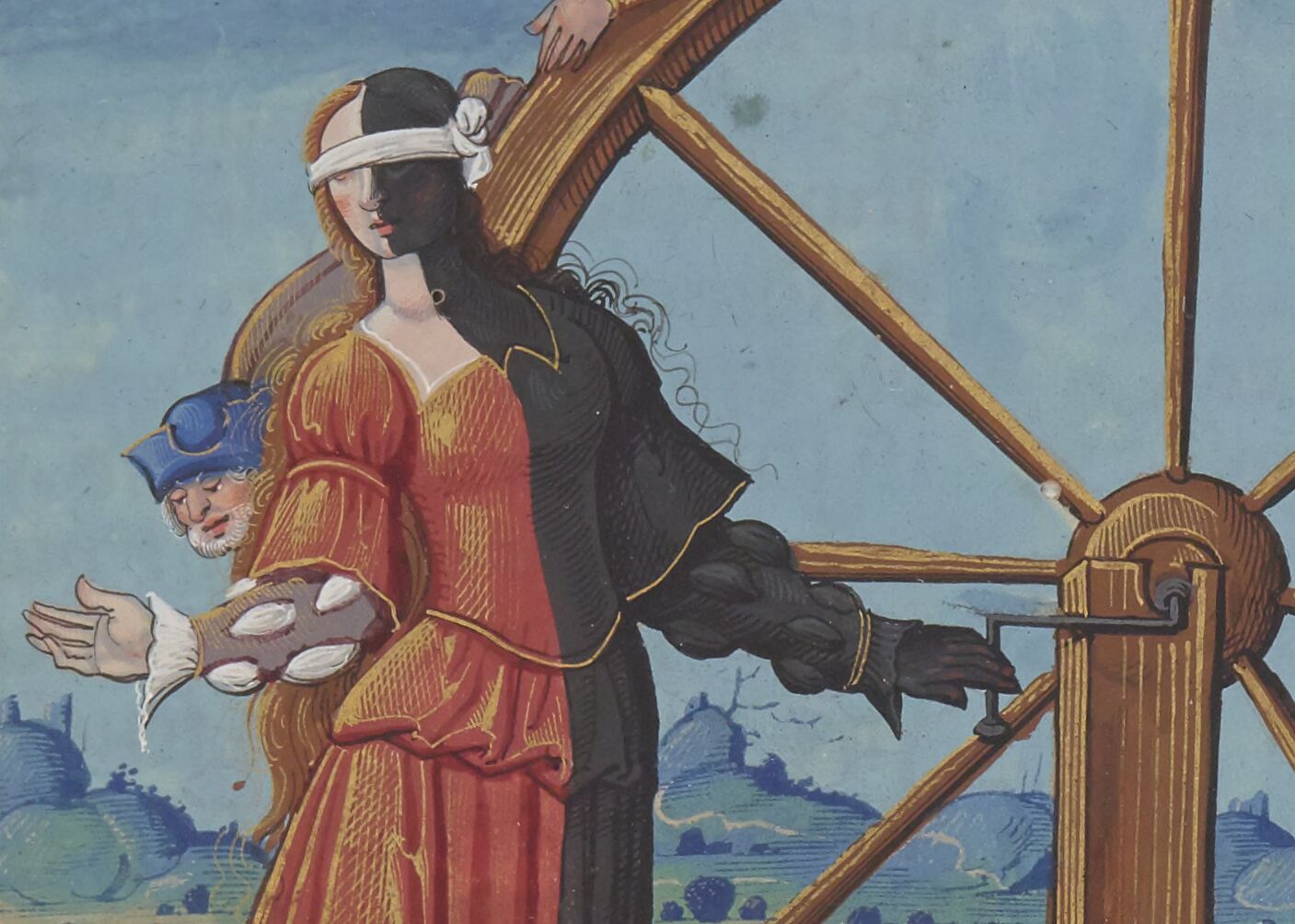This detailed color illustration resembles a scene from a tarot card or a Renaissance-style painting. Set against a backdrop of rolling hills under a blue sky, the focal point is a large wooden wheel in the foreground. A woman stands with her left hand gripping a crank that appears to turn the wheel. Her appearance is a striking personification of duality or good and evil. The left half of her body is entirely black, from the top of her head, through her face and bodice, down to her dress and arm. The right half features rosy-complected skin, red hair, and a reddish-orange dress with a white puffed sleeve and cuff. Notably, her hand on the crank appears normal except for one deformed finger. She is also blindfolded, adding an element of mystery to her identity.

Behind the woman, a man in what resembles a sailor's blue cap peeks over her shoulder, appearing to observe her hand on the crank. Additionally, there are two men strapped to the wheel, suggesting it could be a torture device, although the exact nature of the scene remains ambiguous. The overall impression is an evocative middle-age illustration, rich with symbolism and tightly woven narratives of morality and fate.